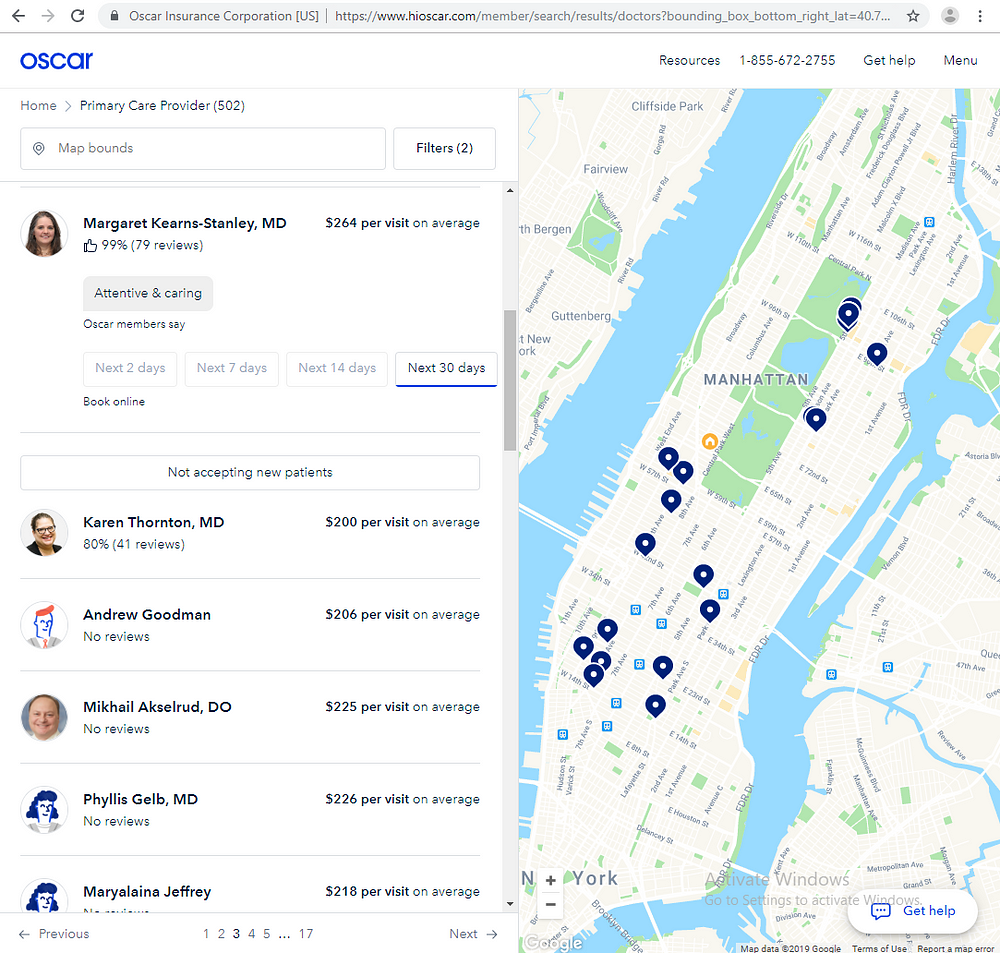This detailed caption describes the layout and content of a web page for Oscar Insurance Corporation's primary care provider search tool. The web page features a map of Manhattan to the right, highlighting multiple physician locations. On the left, the homepage displays primary care provider 502 at the top, followed by a search box for map bounds and filters.

An advertisement prominently features Dr. Margaret Kearns Stanley, MD, whose visits average $264. She is highly rated with a 99% approval rate from 79 reviews and is described as 'attentive and caring.' Buttons below her profile allow users to book appointments within the next 2, 7, 14, or 30 days online.

Below a separating line, the page lists Dr. Karen Tom Thornton, MD, who is not accepting new patients, holds an 80% approval rating from 41 reviews, and charges $200 per visit on average. Next is Dr. Andrew Goodman, with no reviews and an average visit cost of $206, followed by Dr. Mikael Axelrod, whose visits cost $225 on average, also with no reviews. Dr. Phyllis Gelb, MD, appears next with an average visit cost of $226 and no reviews, followed by Marilynne Jeffrey at $218 per visit, though her full profile is not visible.

Navigation arrows for browsing other pages are located at the bottom, with the current page being 3 out of 17. This comprehensive layout allows users to efficiently compare providers, costs, and availability while exploring the map for convenient locations.